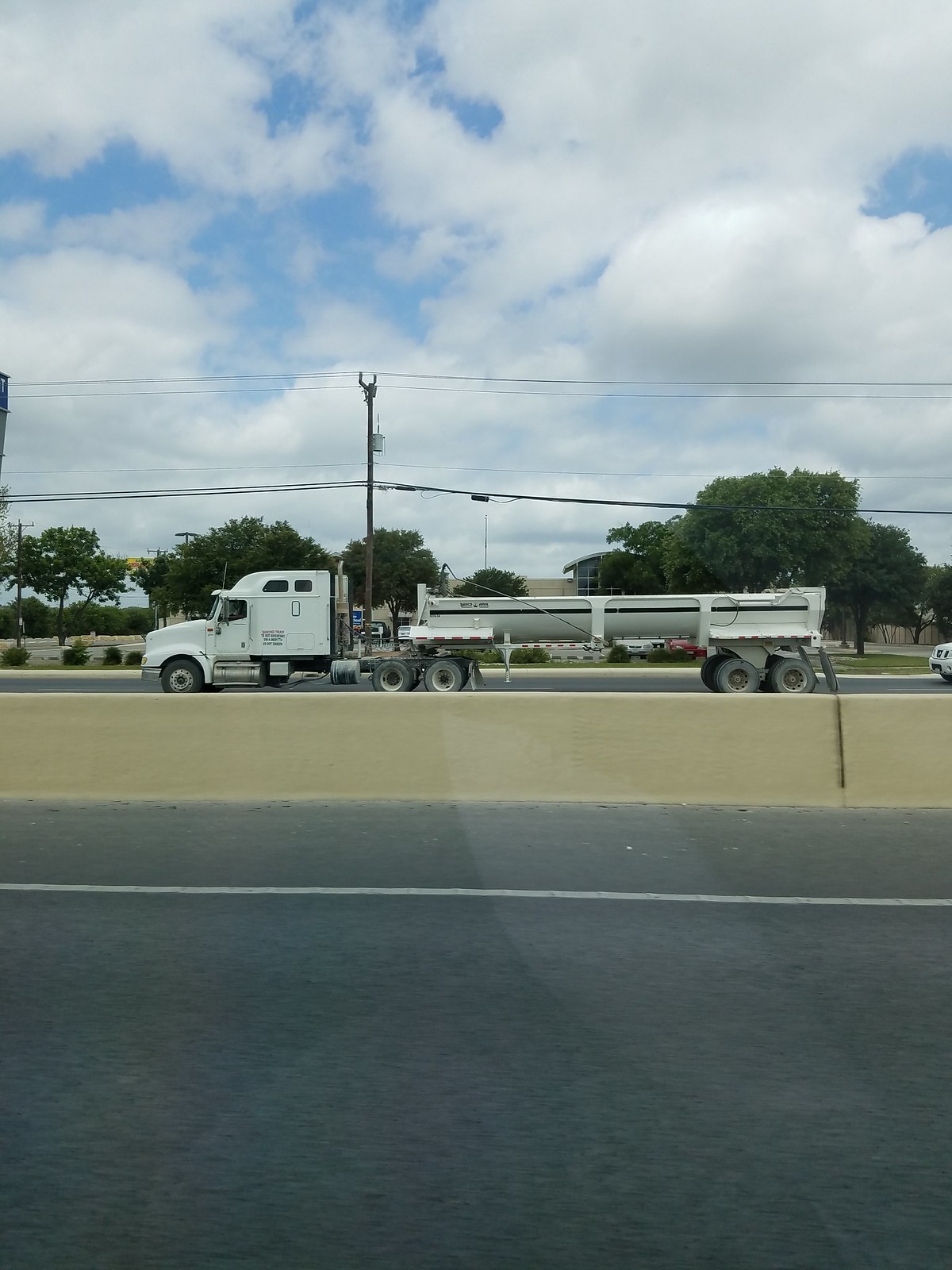This photograph, taken from inside a car, showcases a lively outdoor scene on a highway. The sky above is a light blue canvas punctuated with large, puffy white clouds. Power lines stretch horizontally across the skyline, framing the scene. Below, a lush row of green trees adds a touch of nature to the man-made environment. The highway is divided by a concrete barrier that runs from the left to the right of the image. On the far side of the divider is a wide, open road devoid of traffic, providing a clear view of a large white semi-truck traveling towards the left of the image. The truck's cab is white and it's towing a distinctive trailer that resembles a long, horizontally-cut metal tube. Partly visible behind the trailer is another car, just entering the frame. The reflection off the car window from which the photograph was taken adds a subtle layer of depth to the composition, emphasizing the perspective of the observer. The overall scene captures the intertwined elements of nature and industry under a serene, cloud-dotted sky.